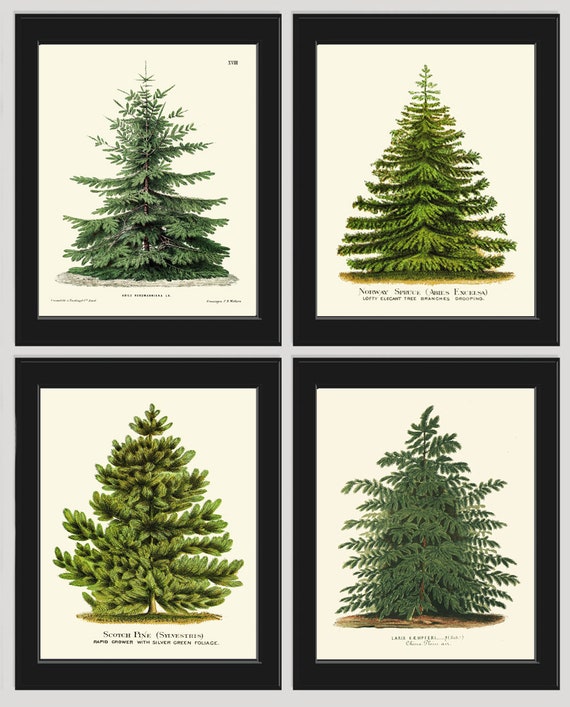The image showcases a set of four framed color illustrations arranged in two rows and two columns, with a slight gap between each. Each frame is rectangular with medium-width black wooden borders, and the pictures are set against a light tan or cream-colored background. The illustrations feature different types of Christmas tree-style trees, each distinctly labeled with black text below the drawings. 

In the top left, there is a short, stocky tree with sparse green needles and spindly branches, presenting a bluish spruce appearance. The tree to its right is the fullest and most classic triangular-shaped tree, characterized by its denser, darker green coat of needles, resembling a long natal pine. On the bottom left is a tree that appears more fern-like with rounded clusters of needles, known as the Scotch Pine, clearly labeled with larger text. Finally, the bottom right tree has a bushy form with a freeform triangular shape and a lighter greenish-blue hue.

These color illustrations are aesthetically consistent, making them an appealing group wall hanging, evocative of various Christmas tree styles.